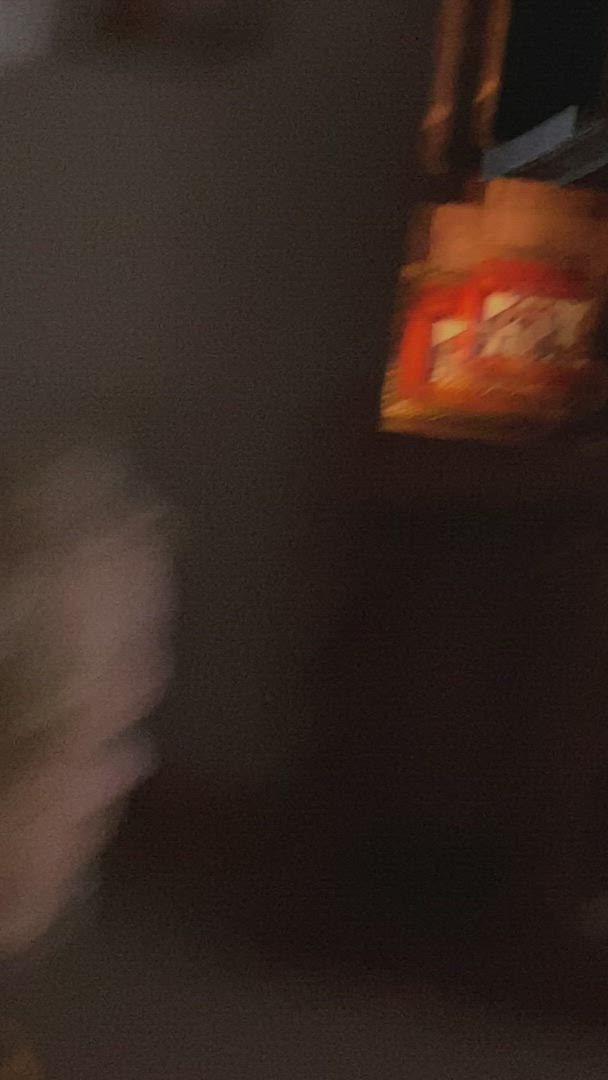This photograph is extremely blurry and dark, making it difficult to discern specific details. The image is a long rectangle, oriented vertically. Most of the photo is black, with a particularly dark area in the center and bottom. In the bottom left corner, there is a vague white or light gray shape that could resemble a face against a white wall. The top right corner features a couple of objects that appear to be barrels or spice jars, characterized by red, plastic-looking rectangles and potentially cork-like tops. They are adorned with some stickers in colors like green and purple, possibly sitting on a countertop. Above these objects, there is a horizontal gray item. The overall photograph appears unsteady and is heavily obscured by darkness and blur.